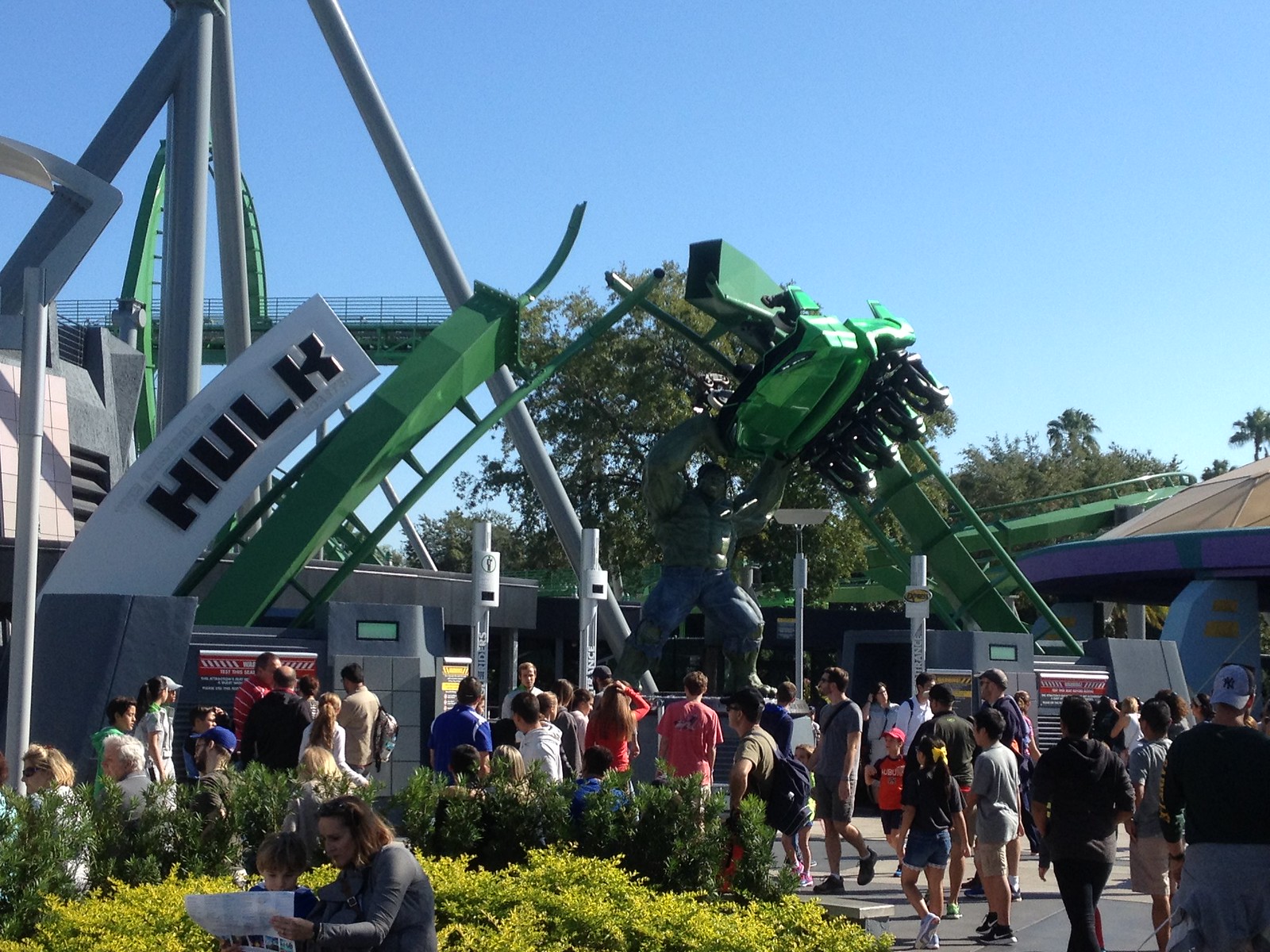This is a detailed daytime photo of an amusement park, likely a Six Flags, featuring the entrance to a thrilling Hulk-themed roller coaster. Dominating the scene is a dramatic statue of the Incredible Hulk, a green, muscle-bound figure dressed in tattered jeans, whose arms are raised above his head as he clutches a green roller coaster car, simulating an intense display of raw power. This eye-catching sculpture serves as an entrance feature, with the roller coaster track appearing broken at the top center where the Hulk grips the car. 

In the left corner of the picture, a woman sits with her son, both engrossed in a map, possibly planning their next adventure. Surrounding the Hulk statue, about 40 excited visitors, both men and women, gaze up in awe at the colossal figure. One man in particular seems to be engaging with part of the crowd, possibly providing information or directions. The backdrop features lush greenery and a few palm trees, enhancing the park's vibrant, lively atmosphere. In the distance, the actual roller coaster, mirroring the design of the entrance display, winds its way through the park, hinting at the thrilling experience awaiting the riders.